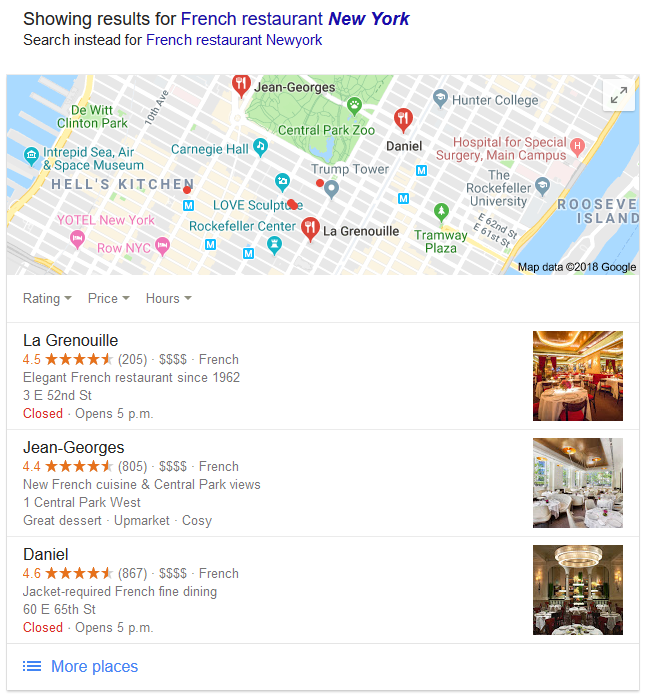Screenshot showcasing search results for "French restaurant, New York" against a white background. The search prompt is highlighted, providing users an option to "Search instead for French restaurant, New York."

The image prominently features a map with several location icons denoting restaurant locations. Additional information such as ratings, price range, and operating hours are provided for the listed restaurants. Three French restaurants are highlighted in detail:

1. **Le Grenouille**
   - *Rating*: 4.5 stars (205 reviews)
   - *Description*: Elegant French restaurant established in 1962.
   - *Address*: 3 E 52nd Street
   - *Hours*: Currently closed (indicated in red), opens at 5 PM.

2. **Jean-Georges**
   - *Rating*: 4.4 stars (805 reviews)
   - *Description*: Features new French cuisine with Central Park views.
   - *Address*: 1 Central Park West
   - *Highlights*: Renowned for its great dessert, upmarket, and cozy ambiance (variant spelling "cosy").

3. **Daniel**
   - *Rating*: 4.6 stars (867 reviews)
   - *Description*: High-end French restaurant requiring jackets.
   - *Address*: 60 E 65th Street
   - *Hours*: Currently closed (indicated in red), opens at 5 PM.

Each listing includes detailed descriptions and user ratings to help diners make an informed choice.